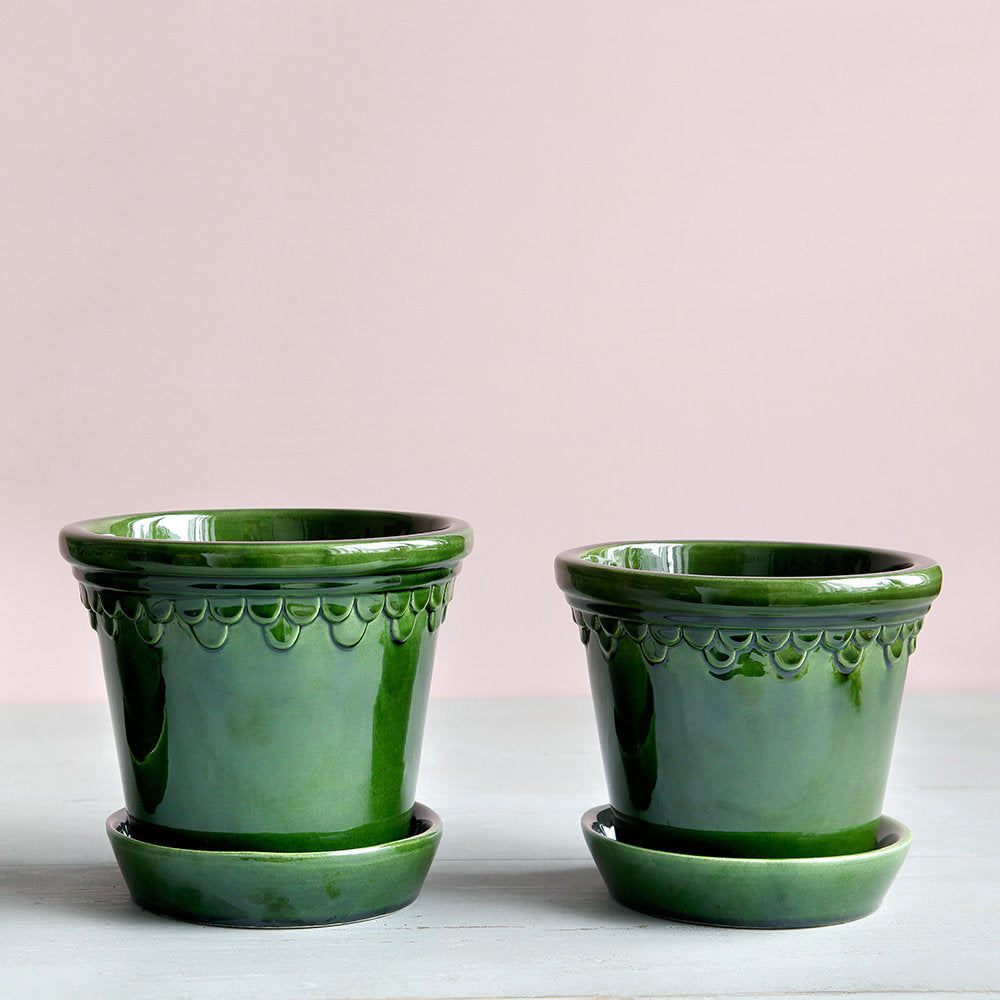The photograph features two ceramic planters set against a pale pink background that gradually transitions into a light blue towards the bottom portion. They are placed atop a whitish table, positioned side by side. Both planters are a medium green color, including their built-in plates, which seamlessly match the pots. The prominent scalloped decorative feature around the rims adds elegance to each planter. Natural light illuminates the glossy green surfaces, creating shadows that extend to the left. The planters are slightly different in size; the one on the left is marginally taller than the one on the right by about one-tenth. This peaceful, square image captures the planters from a frontal point of view, emphasizing their simplicity and subtle sophistication.